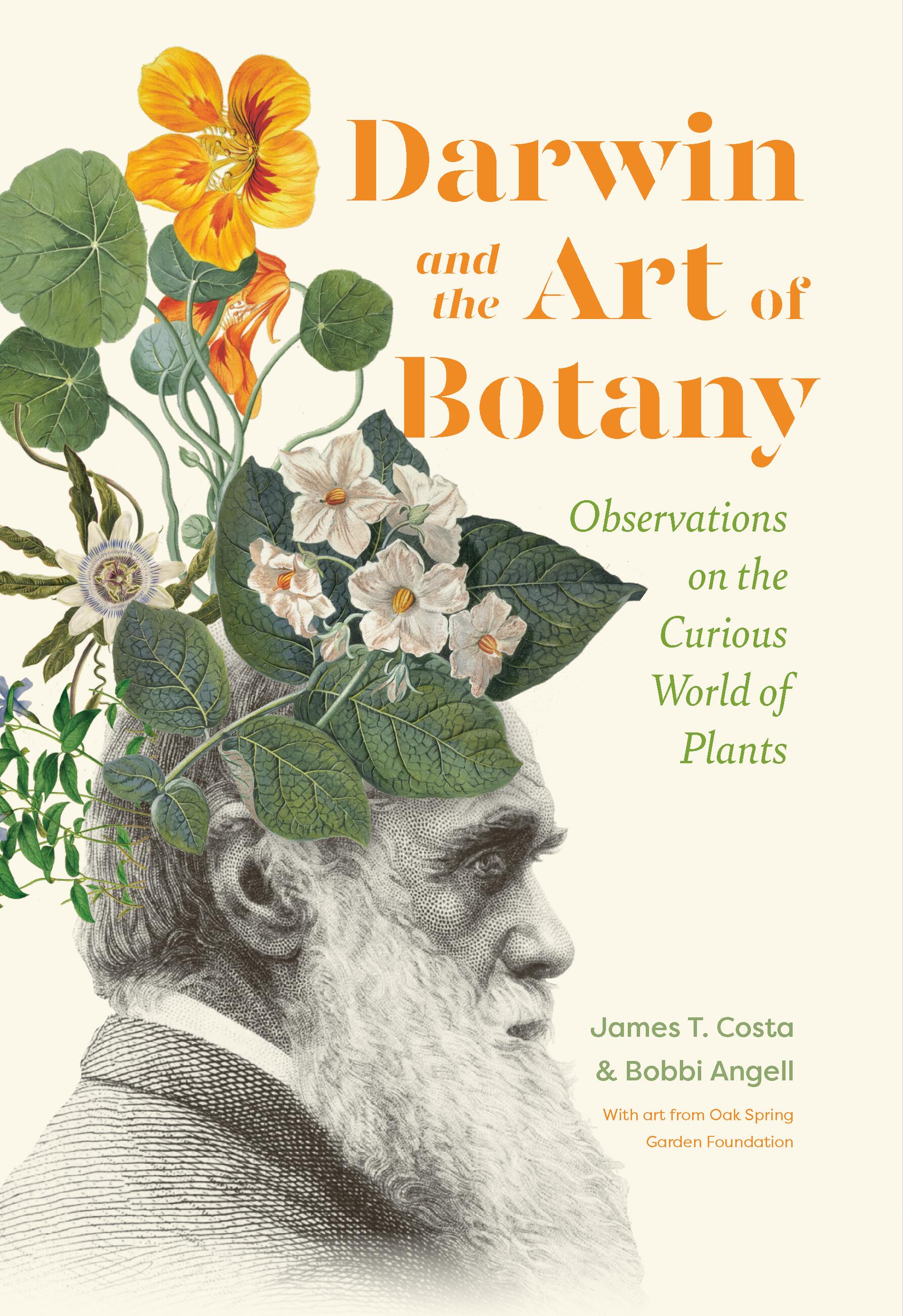A book cover with a light-colored background prominently features a black-and-white illustration of an elderly man with a long, white beard. His face is shaded to bring out his features, and his hair is depicted in varying shades of gray, creating a darker contrast. His eyes appear to be a deep gray. He is dressed in a sport jacket adorned with a checker pattern, paired with a white shirt underneath. The white shirt's collar is visible at the neckline, contrasting against the darker, grayish tones of the jacket. Surrounding the man's head is a lush outcropping of green leaves interspersed with white and yellow flowers, adding a vivid touch of nature to the monochromatic portrait.

The title "Darwin and the Art of Botany" is prominently displayed across the cover in orange letters. Beneath it, in green lettering, reads the subtitle: "Observations on the Curious World of Plants." The author names, James T. Costa and Bobby Angell (spelled A-N-G-E-L-L), are listed in green at the bottom of the cover, followed by a note stating that the artwork is from the Oak Spring Gardens Foundation.